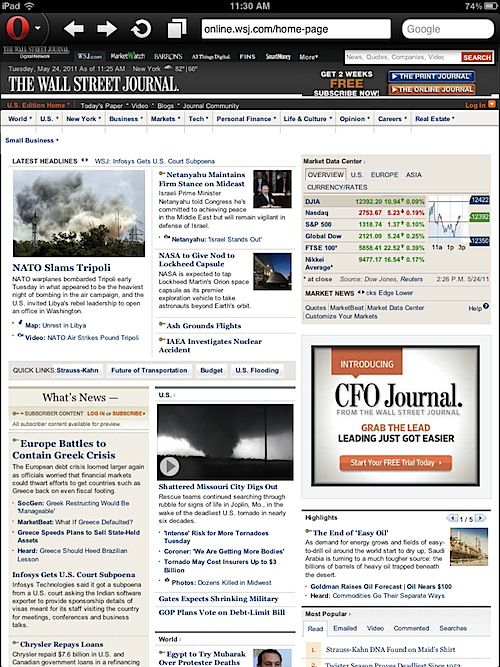This is a detailed screenshot of a Wall Street Journal web page displayed in portrait mode. The top section features a black background with white icons and one distinct red icon resembling a capital "O" situated in the top left corner. A square search bar is prominently positioned in the center, while a rounded rectangle on the top right displays the word "Google."

Below this black banner, the iconic title "The Wall Street Journal" is prominently featured. Just underneath, a navigation bar with various tabs in blue font offers categories such as World, U.S., New York, Business, Markets, Tech, Personal Finance, Life and Culture, Opinion, Careers, and Real Estate. This portion of the page has a contrasting white background.

The content area is divided into three columns. The leftmost column, titled "Latest Headlines," showcases a photograph depicting a fire with significant gray and white smoke billowing into the sky, providing a visual representation of a current news event.